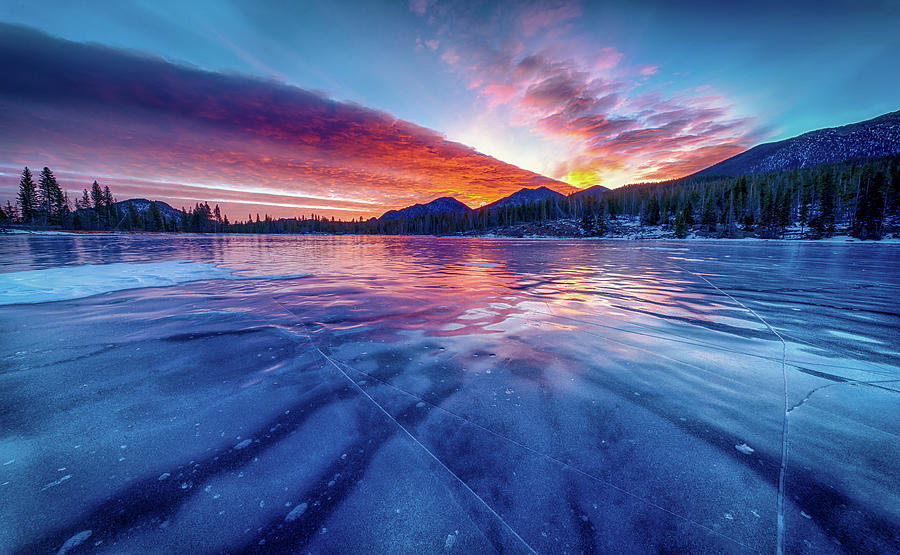This stunning landscape image captures a serene sunset over a large, frozen lake. The smooth, vivid blue ice, crisscrossed with intricate cracks and glistening reflections, dominates the foreground. Within it, patches of white ice add contrast to the vivid sapphire hues. Flanking the ice-covered lake are dense clusters of tall pine trees and snowy terrain. In the background, majestic snow-capped mountains rise against the horizon, their rugged peaks silhouetted against the fading light. The sky above transitions from deep blue to a vibrant tapestry of pink, orange, and amber hues as the sun sets, casting a warm, luminous glow that reflects onto the ice, enhancing the scene’s ethereal beauty.